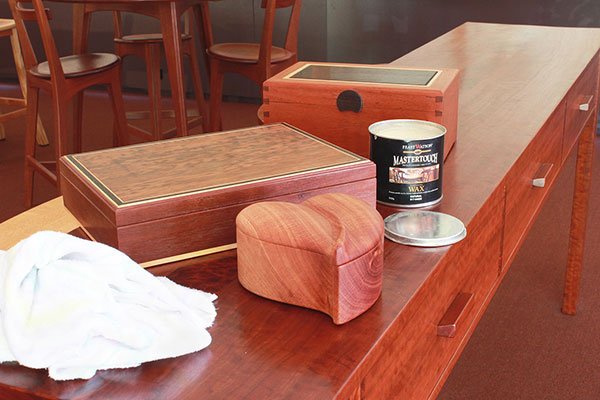This image showcases a long, wooden table with a cherry wood finish, equipped with multiple drawers. The table is topped with a white cloth and three wooden boxes—two rectangular and one heart-shaped. The rectangular boxes exhibit a pronounced wood grain, with one featuring a flat top with a black border and a lighter-colored wood centerpiece, while the taller one has a design reminiscent of a jewelry box. Situated between the two rectangular boxes is an open can of Master Touch wax paint, its contents appearing white. In the background, several solid wood chairs and tables, also in a cherry wood hue, are visible against a brownish floor. A towel rests on the left side of the table, completing the room's cohesive, warm wooden aesthetic.